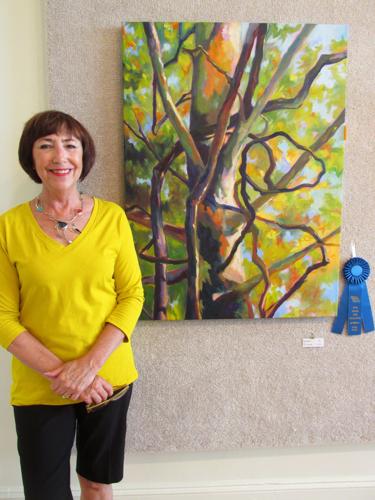In the rectangular photograph, a Caucasian woman with a short brown hairstyle, chin-length, stands on the left side, smiling gently. She is dressed in a bright yellow v-neck shirt with mid-forearm sleeves and black shorts, her hands clasped at her waist, holding glasses in her right hand. Around her neck is a silver necklace adorned with a blue, green, and red pendant. She wears red lipstick, accentuating her radiant smile.

Behind the woman, there is a white wall partially covered by a grey carpet. Mounted on the carpet is a rectangular-shaped painting, presumably created by the woman. The painting is a vibrant depiction of a tree with multiple trunks and entwining vines, with leaves in shades of yellow, orange, and green. The background of the painting includes hues of blue, suggesting a sky. Adjacent to the painting is a blue ribbon with three tassels, indicating that the artwork likely won an award. Below the ribbon, a small placard is visible, further suggesting the significance of the art piece. The woman’s proud and composed demeanor complements the artistic and award-winning atmosphere of the photograph.